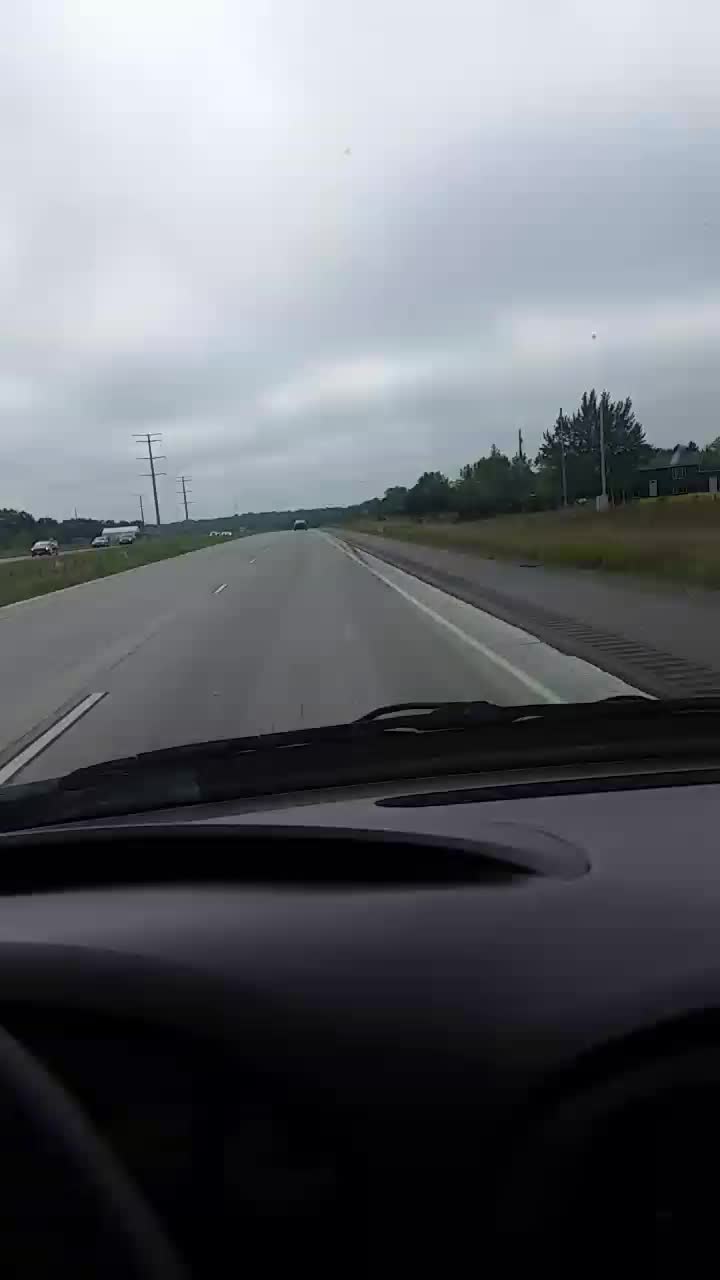Seen through the clear and pristine windshield of a black-interior car, a desolate highway stretches ahead. The black dashboard and a small portion of the black steering wheel are visible in the foreground. The highway, with its freshly paved blacktop, features a solid white line marking the right boundary and a dotted white line delineating the twin lanes. There appears to be a narrow shoulder, potentially a bike lane, flanked by another shoulder equipped with rumble strips designed to alert wayward drivers. Adjacent to the road is a strip of green grass interspersed with tall light poles. In the distance, under a dark and hazy sky tinged with gray and slivers of white, stands a house surrounded by trees.